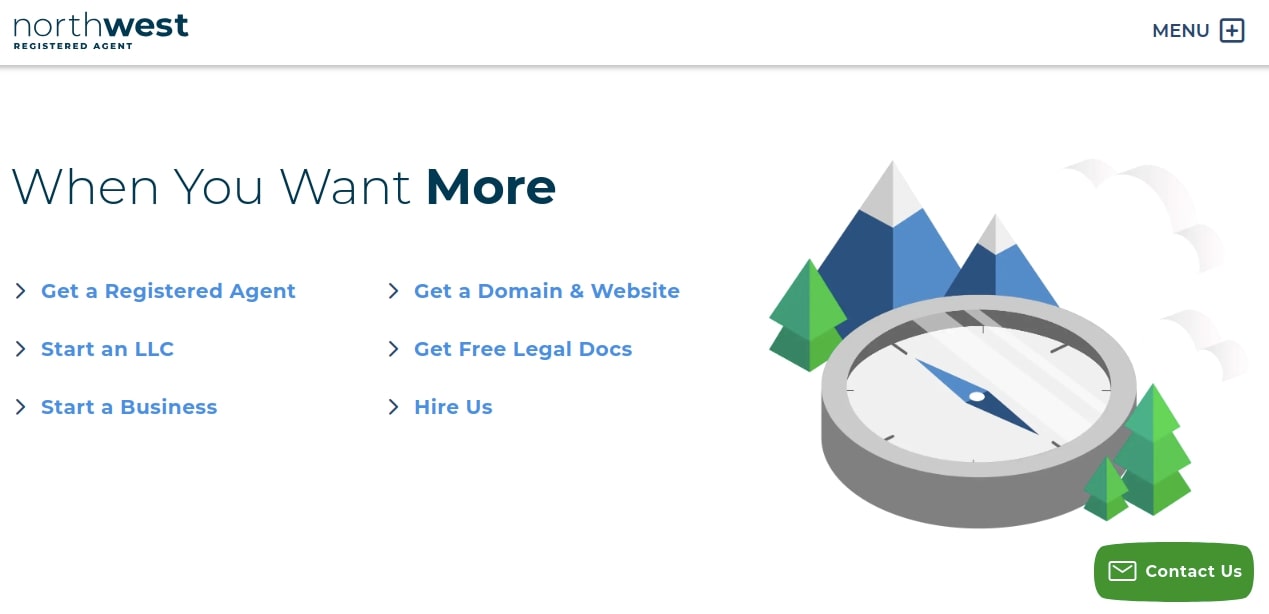The image features a webpage from Northwest Registered Agent, as indicated by the title at the top. Moving towards the right side of the page, a gray line extends from left to right, serving as a divider for the next section. Above this line, on the right, is the word "MENU" displayed in all capital, navy letters. Adjacent to it, there's a navy plus sign inside a white box outlined in navy.

In the middle section of the page, a large font headline reads, "When you want more," with the word "more" presented in bold for emphasis. Below this headline, there are six listed services, divided into three sections on the left and three sections on the right, all presented in a blueprint style. These services include:
- Get a registered agent
- Start an LLC
- Start a business
- Get a domain and website
- Get free legal docs
- Hire us

Each service has an arrow pointing right, indicating more information or a link.

On the right side of the page, a decorative image features black mountains with white peaks, three pine trees, and a compass centered within the scene. Below this imagery is a noticeable green "Contact Us" button, inviting users to reach out.